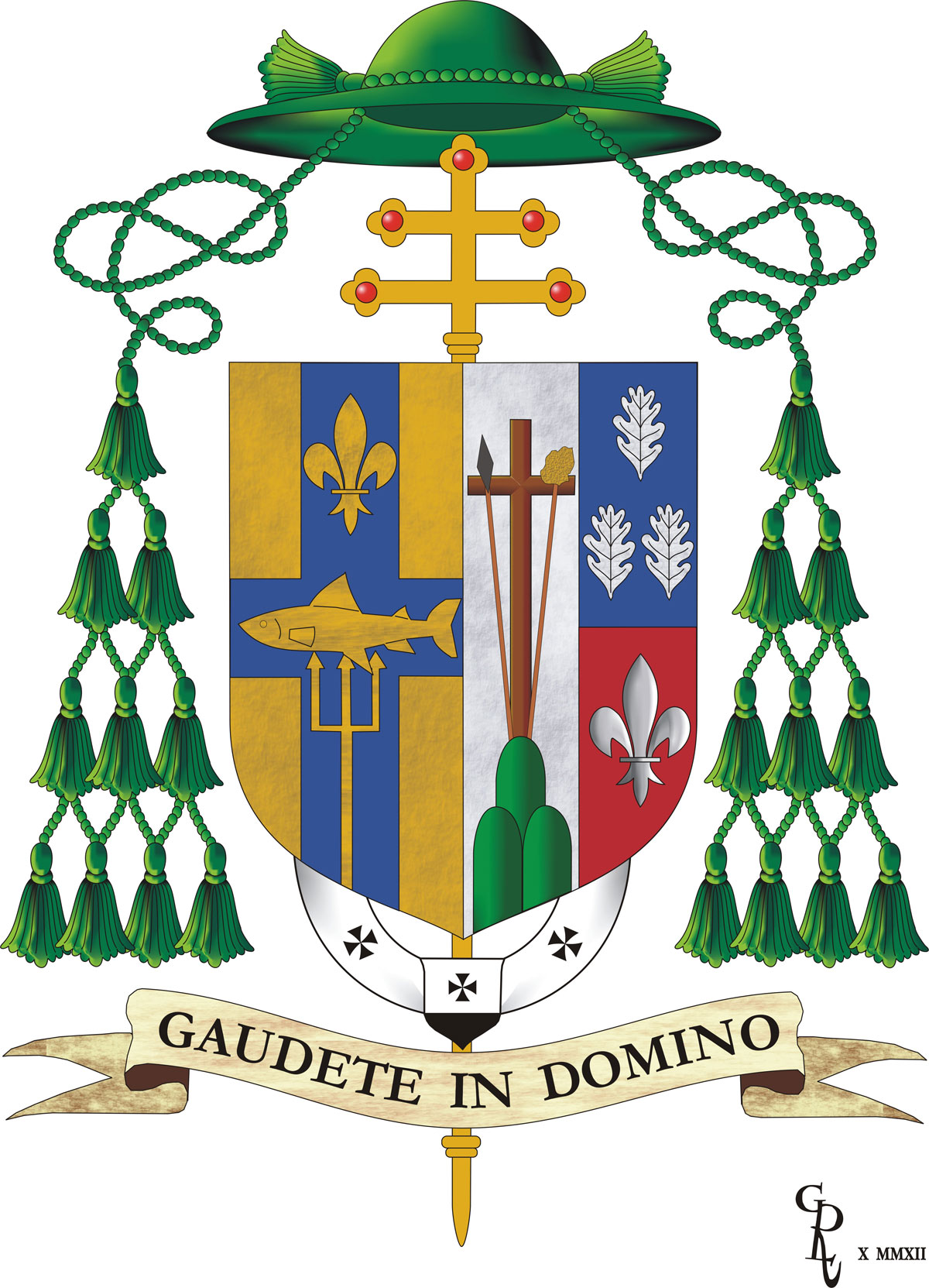The image is a detailed computer-generated depiction of a family crest against a solid white background. At the top, there's a wide-rimmed green bonnet adorned with tassels. These tassels cascade symmetrically down both sides, culminating in ten smaller green tassels arranged in a triangular formation—one at the top, followed by two, three, and then four at the base.

In the center of the image sits the shield-like crest, divided into two distinct halves. The left half features a gold background with a prominent blue cross. Embedded within this cross are three elements: a gold trident at the bottom, a gold fish in the middle, and a three-leaf design at the top. 

The right half of the shield is segmented into three parts. The upper section is blue with white leaves, the middle section is white with a brown cross and three green ovals at the bottom, and the lower section is red with additional white leaf motifs. Below the crest, written on a cream-colored ribbon with black text, is the phrase "Gaudet in Domino."